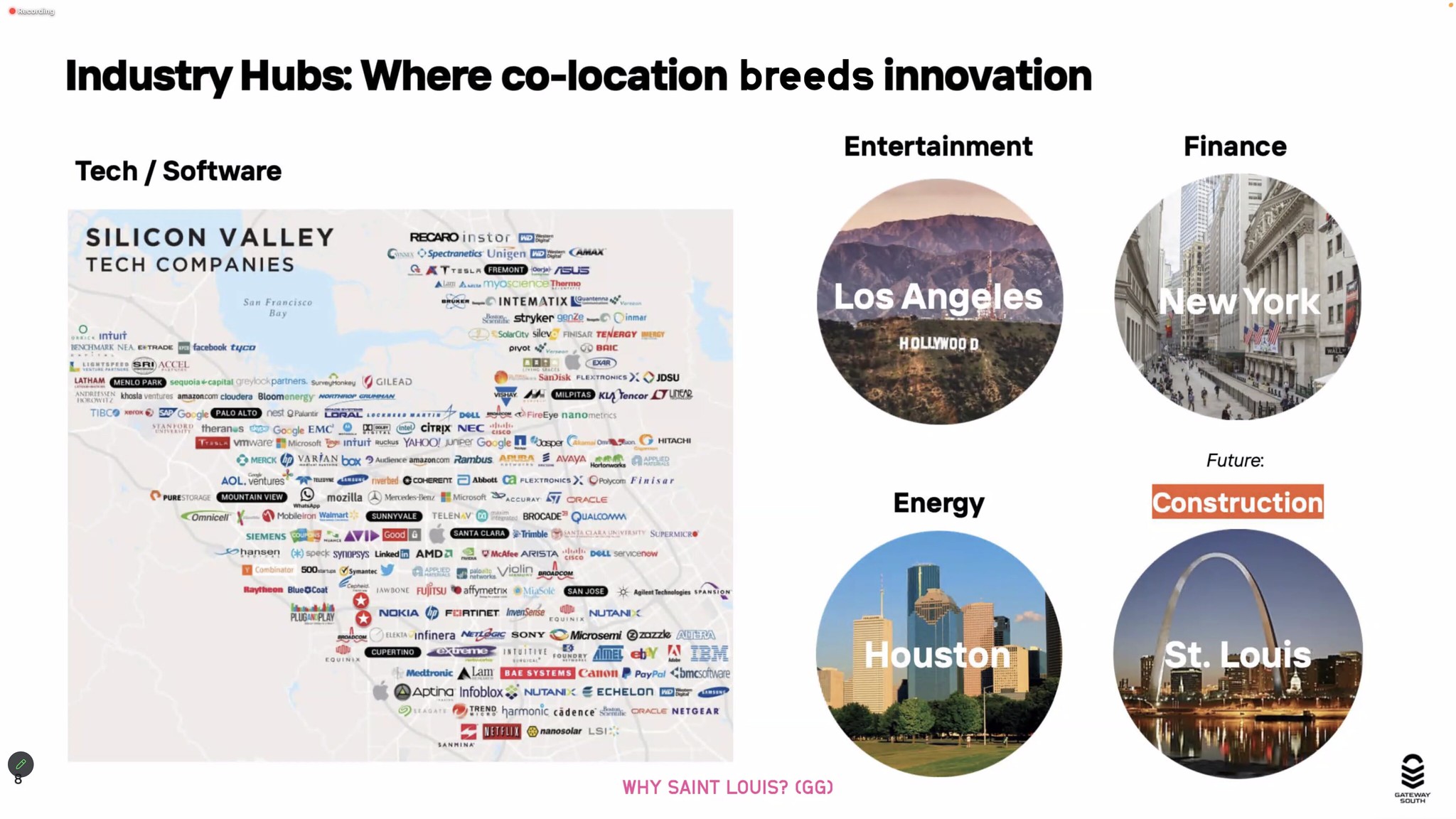The image features a predominantly black and white chart titled "Industry Hubs: Where Co-location Breeds Innovation," emphasizing the collaborative potential of companies working together. Dominating the left side is a map, while the upper left showcases a detailed section on Silicon Valley Tech Companies, listing numerous tech firms such as AMD and Intimatex. To the right, four distinctly colored and labeled circles represent major industry hubs: Los Angeles for entertainment, highlighted by the iconic Hollywood sign and purplish mountains; New York for finance, depicted with city skyscrapers; St. Louis for construction, marked by its gleaming arch and an orange banner stating "future construction"; and Houston for energy, featuring its skyline and park. The image concludes with the phrase "Why St. Louis?" in pink. The overall color scheme is primarily white and black, with additional colors accentuating significant elements.